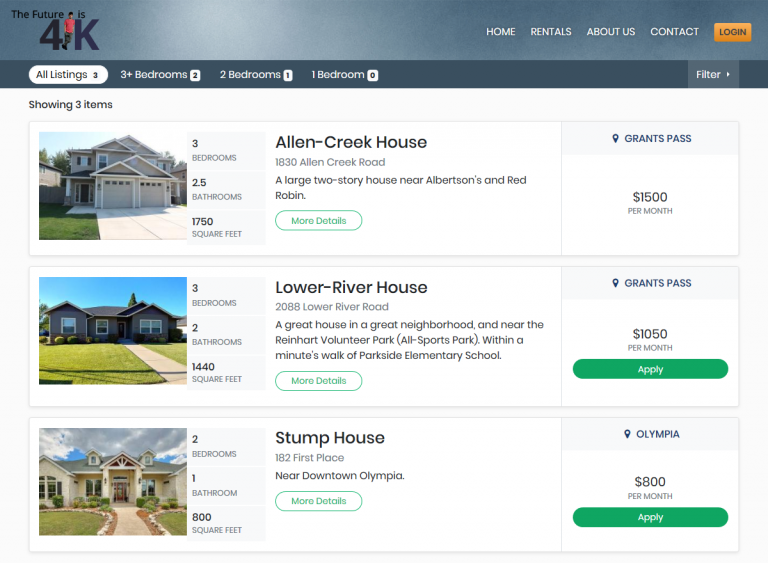This screenshot displays a real estate webpage with a large, prominent title bar occupying the top two-thirds of the image. The background of the title bar features a medium blue color with lighter blue highlights. On the left side of this section, the words "The Future Is" are written in black text. Directly below, a larger numeral "4" is placed next to a stylized figure of a person with short black hair, medium-toned skin, wearing a red short-sleeved shirt, gray pants, and black sneakers. The figure is leaning on a capital letter "K."

To the right, the top navigation menu showcases five categories in white all-capital letters against the blue background: "HOME," "RENTALS," "ABOUT US," and "CONTACT." An orange box with black text on the far right says "LOGIN."

Underneath this main bar, a darker blue horizontal line features several search filter options in a rounded white rectangle with black text. It starts with "ALL LISTINGS" followed by the number "3." Adjacent to this, in white text against the dark blue background, are the options "THREE+ BEDROOMS" with a small white box containing the black number "2," "TWO BEDROOMS" with a small white box containing the black number "1," and "ONE BEDROOM" with a small white box containing the black number "0." The far-right of the dark blue line displays a medium gray box with white text that reads "FILTER," accompanied by a small right-hand arrow.

Below the title and filter sections, the page presents three real estate listings. Each listing includes details about the city location and the monthly rental cost for each home.